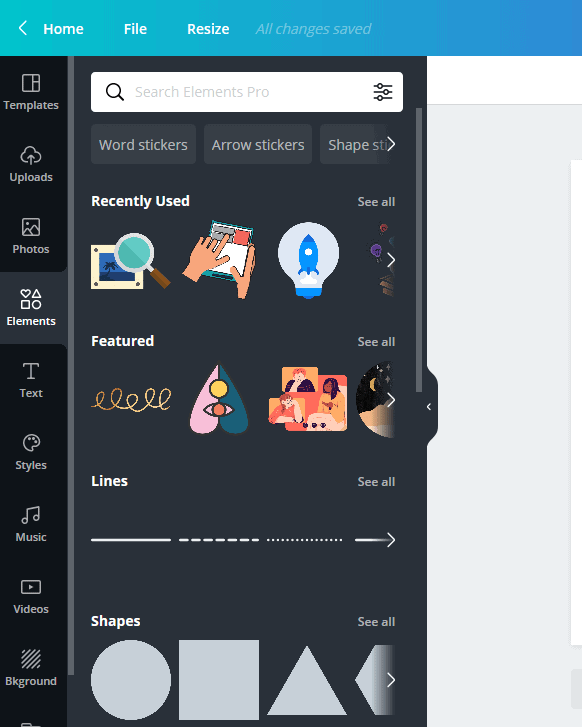Screen capture of a graphical user interface, likely from an application on an iPad or computer. The interface features a top ribbon with three visible tabs labeled "Home," "File," and "Resize." A message indicating "All changes saved" appears shaded out. Below the ribbon, the left column contains a series of icons with accompanying labels: Templates, Uploads, Photos, Elements, Text, Style, Music, Videos, and Background.

To the right of this column, an expanded window displays the "Elements" section, highlighted in the left column. At the top of the expanded window is a search bar. Below the search bar, there are sections for "Word Stickers" and "Arrow Stickers," followed by a row of "Recently Used" items. The recently used items feature colorful icons, including a search icon and a light bulb with a rocket inside it.

Lower in the expanded window, a "Featured" row displays unique icons such as a squiggly line, an upside-down heart, and a collage of graphics. Further down, the interface provides a section for "Lines," offering various types such as straight, dashed, and dotted lines. At the bottom, the "Shapes" section includes icons of a circle, square, triangle, and octagon, all presented in colorful designs.